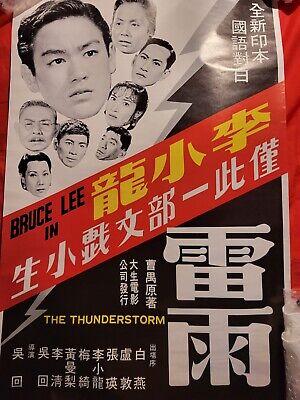This appears to be a detailed movie poster for one of Bruce Lee's early films titled "The Thunderstorm." The poster is predominantly in Chinese, featuring a mix of yellow and white characters. At the top left corner is a large black and white image of Bruce Lee's head, alongside the faces of seven other individuals, possibly co-stars, also presented in black and white. These faces are set against a white background, and most of the individuals have dark or graying hair, with one wearing glasses.

A striking red diagonal banner cuts across the middle of the poster, prominently displaying the text "Bruce Lee in" in black letters. Above this banner, yellow Chinese characters are visible, followed by a column of white Chinese characters. The bottom section of the poster features more white characters as well as the movie's title, "The Thunderstorm," which is emphasized in bold yellow text. Additionally, there are silver or gray jagged lines, resembling lightning bolts, one of which runs down the right side, aligning with the movie's title theme. In the bottom-right corner, there appear to be white stacked objects that look like cups. Overall, the poster conveys a sense of dramatic intensity, reinforced by its bold graphics and storm-related imagery.